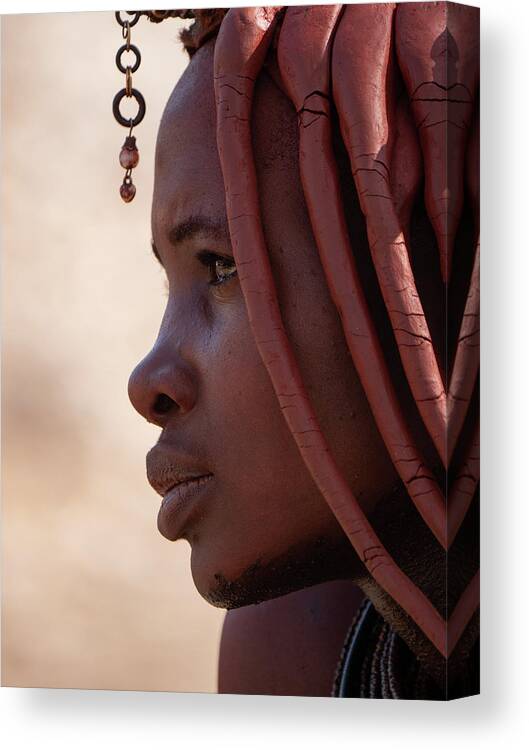This professionally captured photograph, printed on a vertically rectangular canvas without a distinct border but with shading on the left and lower portions, features an African gentleman in profile, facing left. The image utilizes natural daylight, lending a vibrant and authentic ambiance to the scene. The background is blurred with a blend of reddish and whitish hues, which heightens the focus on the subject.

The man’s hair is intricately styled into thick braids enveloped in a reddish mud, giving his hairstyle a solid, sculpted appearance reminiscent of traditional cultural practices. A barely visible necklace peeks from the lower right corner of the frame, adding a subtle accent to his attire. On his forehead, a delicate piece of forehead jewelry adorned with small red beads extends just above his eyebrows, contributing to his dignified and thoughtful look. The composition and details emphasize the cultural richness and personal expression of the individual, enhancing the overall depth and meaning conveyed through the portrait.